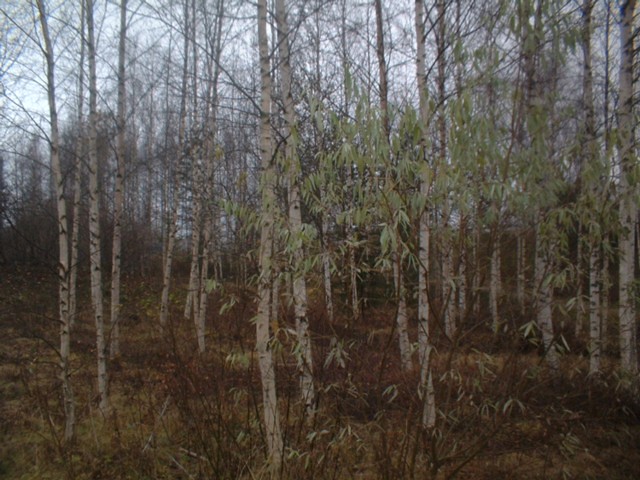The photograph captures a serene wooded area during daytime, characterized by an array of tall, thin trees with almost white bark. The trees, mostly bare with very small, sparse leaves, stand amidst a brownish, seemingly lifeless ground interspersed with some weeds. The image is rectangular, wider than it is tall, featuring a foggy, grayish blue sky peeking through the barren branches, suggesting a hazy atmosphere. In the foreground, particularly on the left and right sides, a secondary type of flora resembling spindly vines with long, narrow, light green leaves climbs upwards. The forest floor varies in color from light tan to darker brown, covered in sparse shrubbery and adding to the overall muted, tranquil ambiance of the scene.